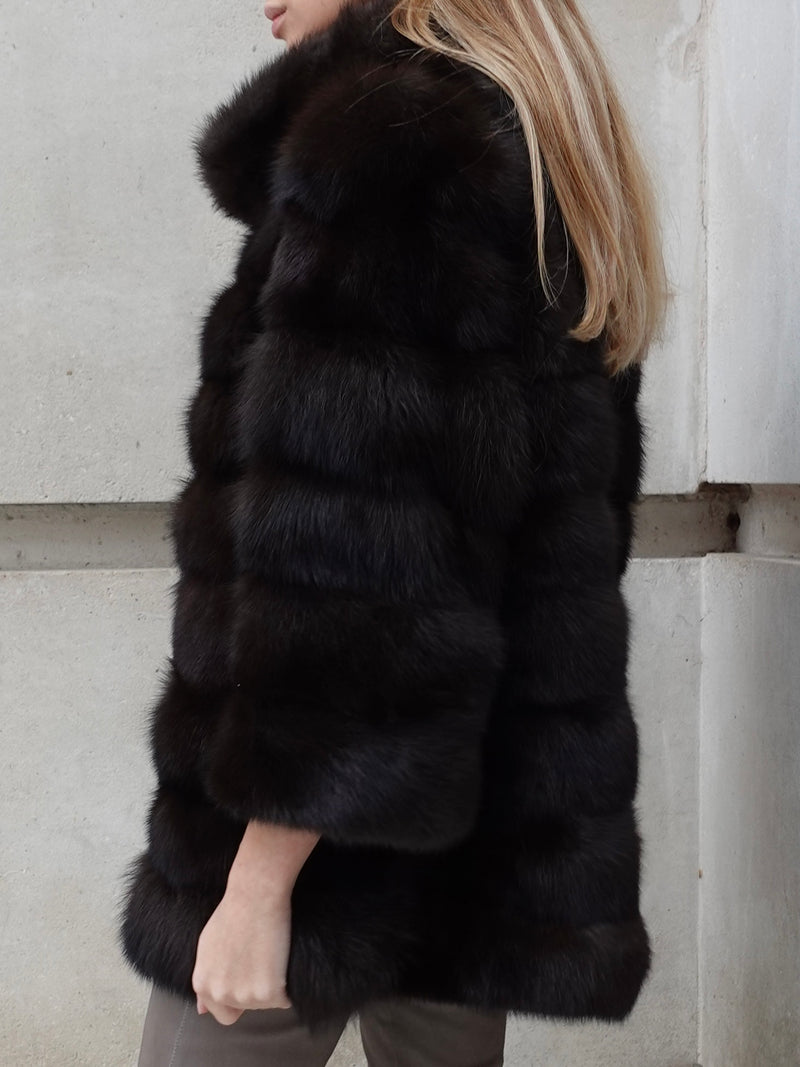A stylish woman stands outdoors, wearing a luxurious thigh-length black fur coat with a fuzzy texture and horizontal ridges along its body and sleeves. The coat has wide sleeves that end just before her left wrist, and she's facing to the left, only the bottom third of her face visible, showcasing her lips and long, striated blonde hair cascading down her back. Just a glimpse of her light gray pants is visible beneath the coat. In the background, there's a gray stone or concrete wall with a darker horizontal channel that runs across the middle, adding a contrasting architectural element to the image. Her left hand hangs naturally at her side, accentuating the coat's plush elegance.